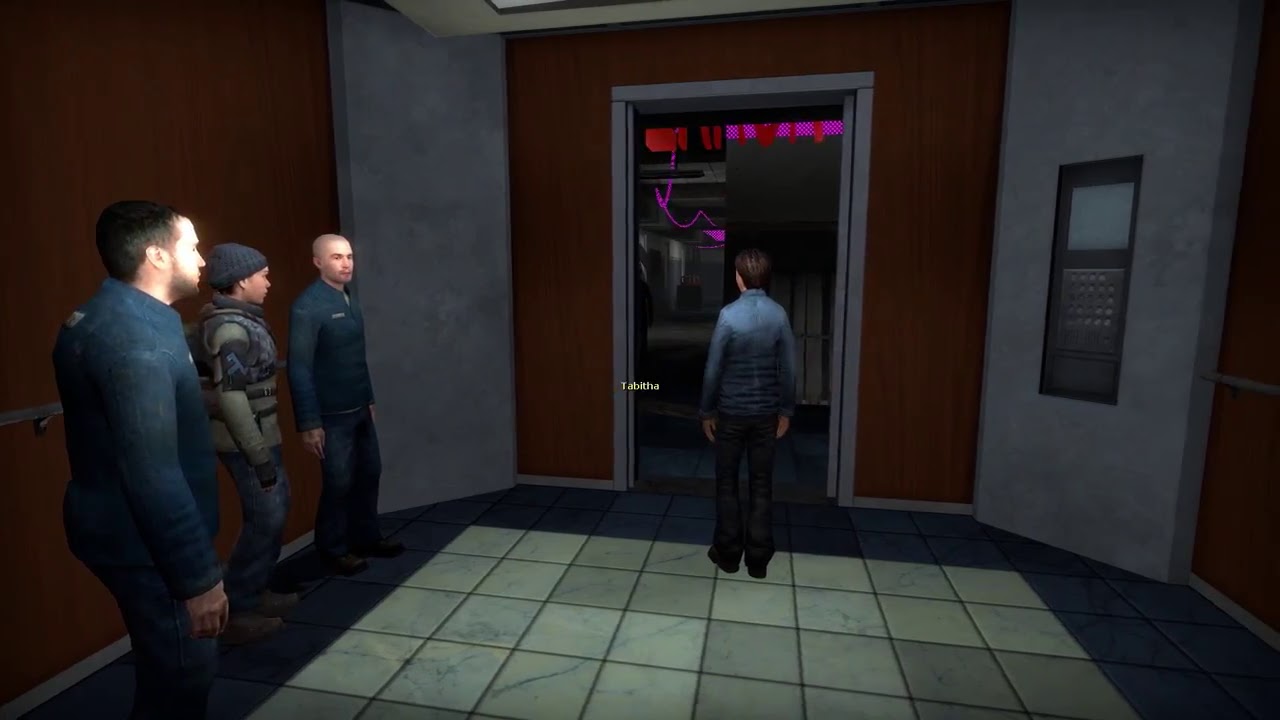The image is a dark, nighttime screenshot from a video game depicting a small, dimly lit room with a tiled floor and alternating dark red and gray walls. In the center, we see a character with their back to the camera, wearing a blue top and black pants. Above their head, the name "Tabitha" is displayed in white letters. This character appears to be about to walk through an open doorway, which features a keypad-like device with a screen, reminiscent of an ATM or code panel, on the right-hand side.

To the left of this central figure, three other characters are visible. Two of them, males in navy coveralls, stand alongside a third character who appears to be a woman. One of the men is distinguishable by a ski cap and what looks like a bulletproof vest or armory. The room is dark, making it difficult to discern finer details, but an array of purples and reds in the image contributes to its overall shadowy atmosphere.